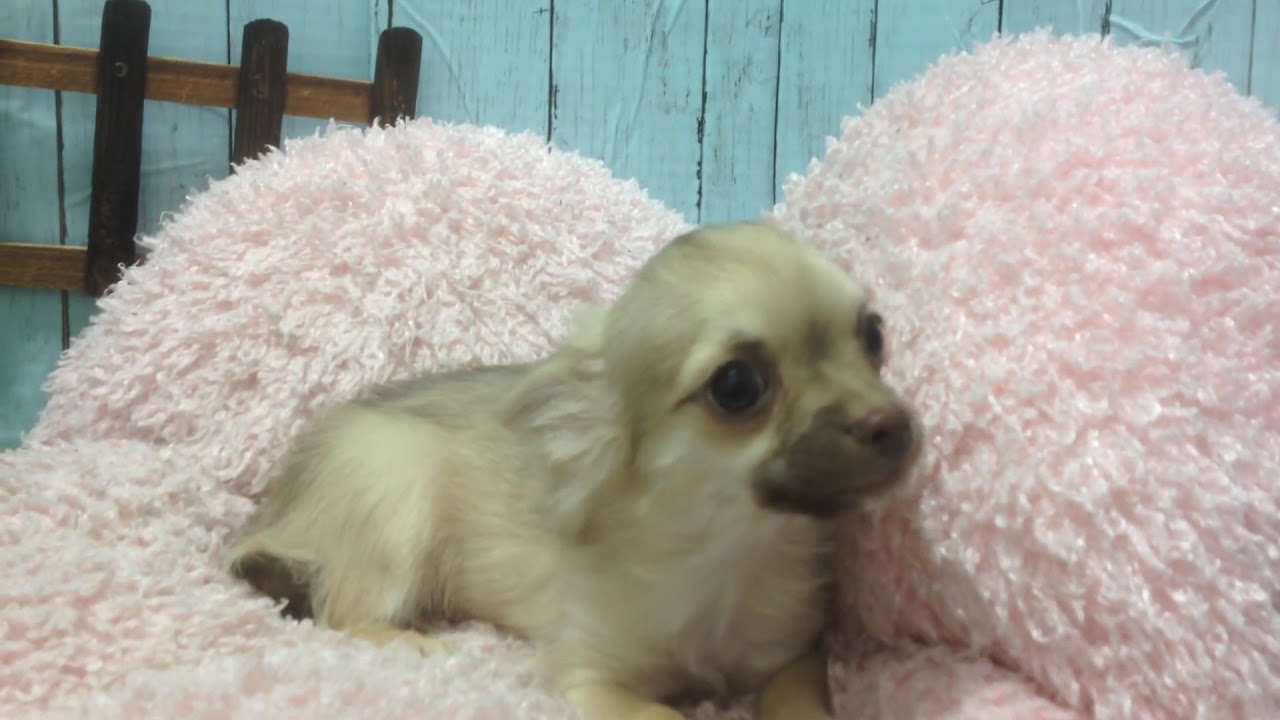The image features an adorable, tiny Chihuahua or Chihuahua mix puppy with medium-length, cream-colored fur, resting on a soft, fluffy, heart-shaped pink pillow. The dog has large, bright brown eyes and a small brown nose, with some darker brown fur around its mouth. Its ears are set back as it looks curiously to the right, away from the camera. The pillow, significantly larger than the puppy, forms two mounds on either side of it. The background showcases a pale blue, wooden wall with boards of varying sizes. On the left side of the image, there's a simple, wooden decorative fence or headboard adding a rustic touch to the scene.